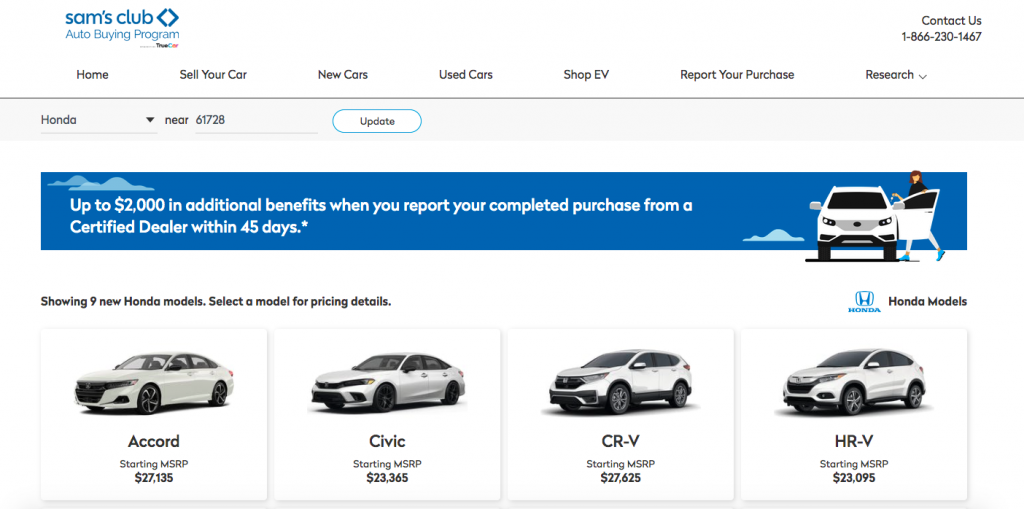The image showcases the Sam's Club Auto Buying Program interface. The top left corner prominently displays the program name in blue lettering along with its logo, and just below it is the smaller Truecar logo. In the top right corner, "Contact Us" and a phone number are provided for assistance. Below this section, a navigation bar features clickable fields including Home, Sell Your Car, New Cars, Used Cars, Shop EV, Report Your Purchase, and Research, all in black text against a white background.

Beneath the navigation bar, there is a drop-down menu to select the make of the vehicle you're searching for, alongside a field to enter your zip code. Accompanying this section is an update button outlined in blue. Positioned centrally on the page is a deep blue banner with white lettering that announces, "Up to $2000 in additional benefits when you report your completed purchase from a certified dealer within 45 days." To the right of this banner is a small illustration of a woman entering a car.

Further down, the page displays four vehicles listed for sale, under a heading that reads, "Showing nine new Honda models. Select a model for pricing details." The models showcased include the Accord, Civic, CR-V, and HR-V, each with their respective prices listed below the images.